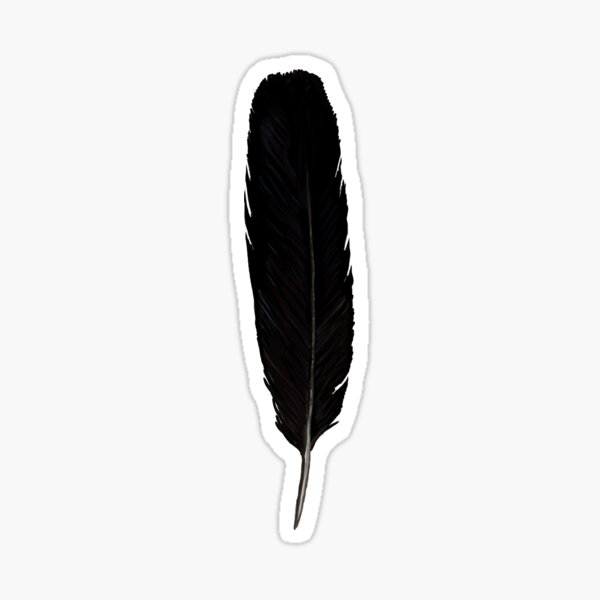This image features a black, hand-drawn feather resembling a quill, prominently centered against a gray background. The feather is accentuated by a distinctive white border which helps it stand out, much like a sticker one might find on Redbubble. The feather's shape and detailing evoke a traditional ink pen used for historical signatures, such as that of the Declaration of Independence, with the shaft of the feather running vertically from the sharp lower tip to the top. The feather appears thick with intricate lines, and though the central line is slightly uneven, each edge of the feather shows individual strands clearly. The overall image sits within a slightly rectangular, portrait-oriented frame, maintaining a minimalistic and artistic aesthetic.